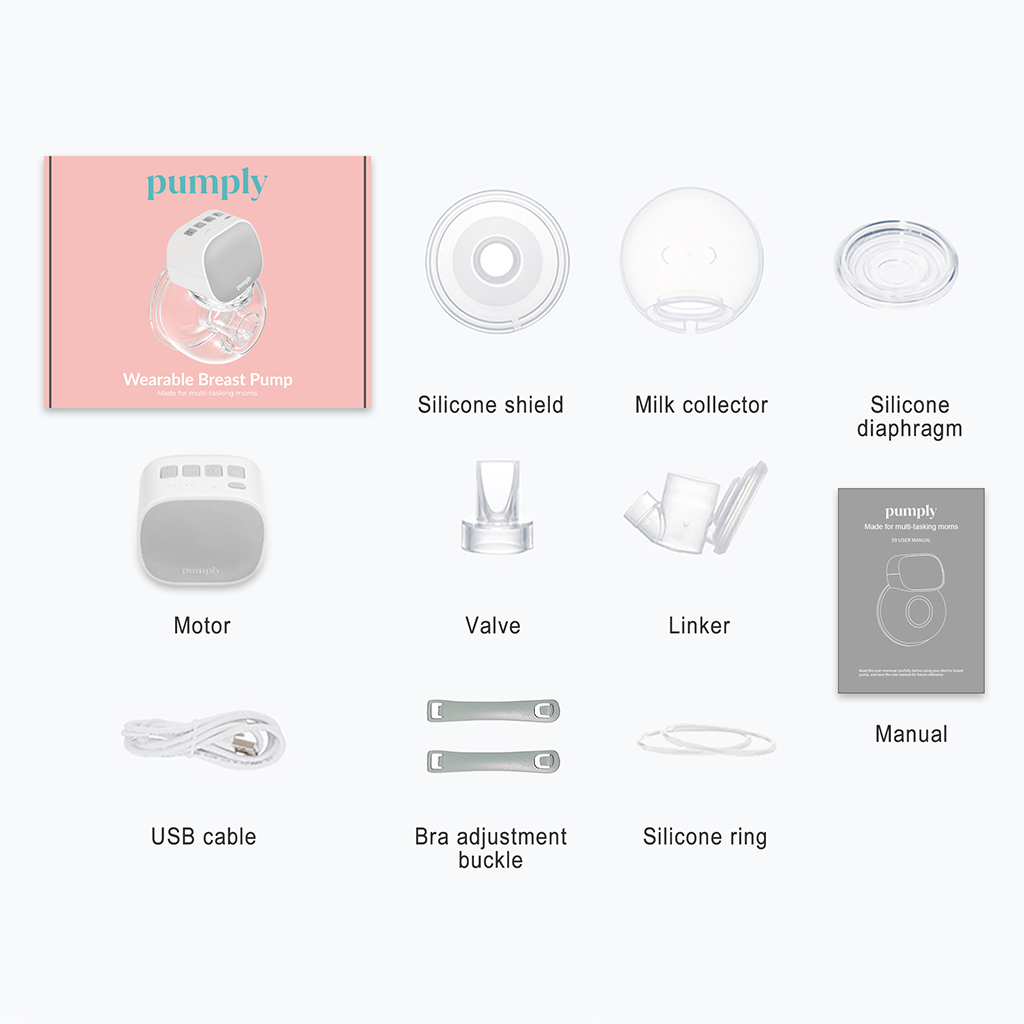This detailed image presents the contents of a "Pumply" wearable breast pump box, arranged meticulously against a white background. Positioned in the top left is the "Pumply" box, characterized by its distinct pink color. Adjacent to the box are images of each component included inside. 

Starting from the top, the arrangement showcases a silicone shield, designed for comfort and optimal fit during use. Next, we have a milk collector, a circular vessel essential for collecting expressed milk. Below it, there is a silicone diaphragm, which operates as part of the pump mechanism. 

Also included is the motor, a compact, whitish-gray device that powers the breast pump. The collection continues with a valve that regulates milk flow, a linker which connects the various components, and a USB cable, a white cord neatly zip-tied, used for recharging the motor.

Additional accessories include a bra adjustment buckle for enhanced fit and support, a silicone ring presumably for securing parts together, and finally, an instruction manual. This manual, a gray booklet with the "Pumply" branding on its cover, provides comprehensive guidance on operating the breast pump.

Each item is individually photographed to highlight their form and function, providing a clear overview of what users can expect upon unboxing their Pumply wearable breast pump.